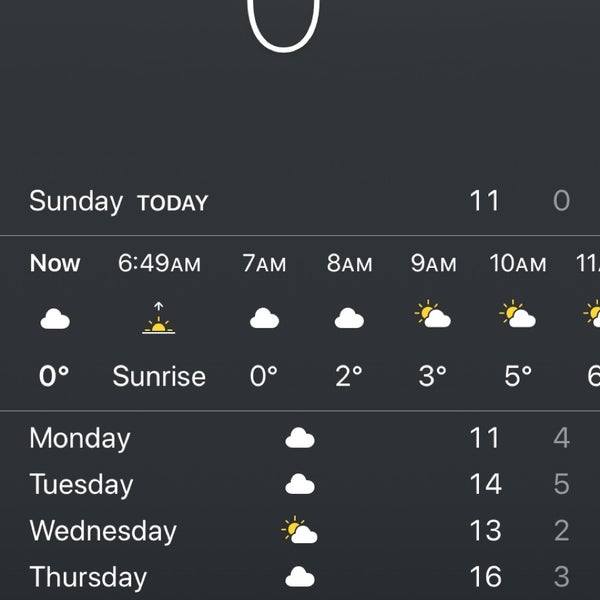A colour screenshot displays a segment of a weather app on a smartphone or tablet. The interface features a sleek black background with contrasting white text. At the top centre, an incomplete number is visible, appearing to be the bottom half of a zero. Below this, the text reads "Sunday" followed by "Today" with a series of numbers: 11 on the right side and a zero directly beneath it.

The interface then transitions to a timeline, starting with "Now" and progressing through incremental times: 6:49 AM, 7 AM, 8 AM, 9 AM, 10 AM, and 11 AM. Next to "Now," a cloud icon is displayed, indicating current weather conditions. At 6:49 AM, the text "Sunrise" is noted. The temperature readings follow: "Now" at 0 degrees, 6:49 AM at sunrise, 7 AM with a cloud icon and 0 degrees, 8 AM with a cloud icon and 2 degrees, and 9 AM with partial clouds and sun at 3 degrees. The pattern continues with 10 AM being partially cloudy at 5 degrees, and 11 AM showing partial clouds with approximately 6 degrees (last digit is slightly cut off). Thin horizontal white lines delimit these sections.

Further down, there's a 4-day forecast featuring: “Monday,” “Tuesday,” “Wednesday,” and “Thursday” aligned on the left. Icon summaries display cloud icons for Monday, Tuesday, and Thursday, while Wednesday shows partially cloudy conditions. Each day includes minimum and maximum temperature readings: Monday (11/4), Tuesday (14/5), Wednesday (13/2), and Thursday (16/3). The temperature units are not explicitly mentioned, leaving it unclear whether they are in Celsius or Fahrenheit.